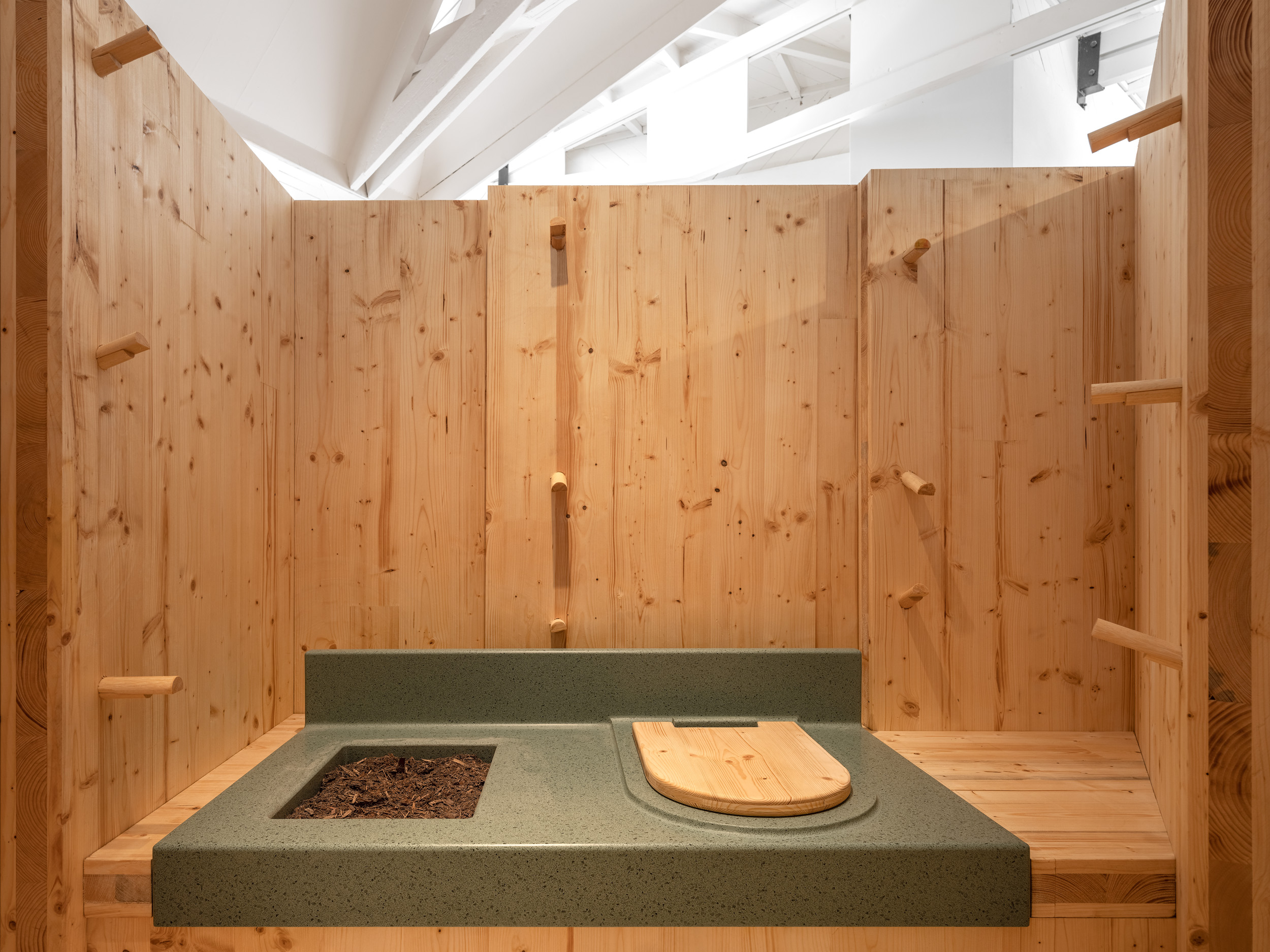This image depicts an unconventional and clean outhouse setup, possibly displayed at a trade show or convention hall, given the white interior and large metal beams visible overhead. The primary components include a green plastic base set atop a wooden platform, with a wooden toilet lid resembling those found in porta-potties. Alongside the sitting portion of the toilet, there is a small dirt pit, likely intended for standing use. This setup is surrounded by wooden walls that exhibit a light brown or tan wood grain, and from these walls, numerous wooden pegs protrude. The entire structure is roofless, enhancing the visibility of the convention hall's white-painted beams and the spacious indoor environment.